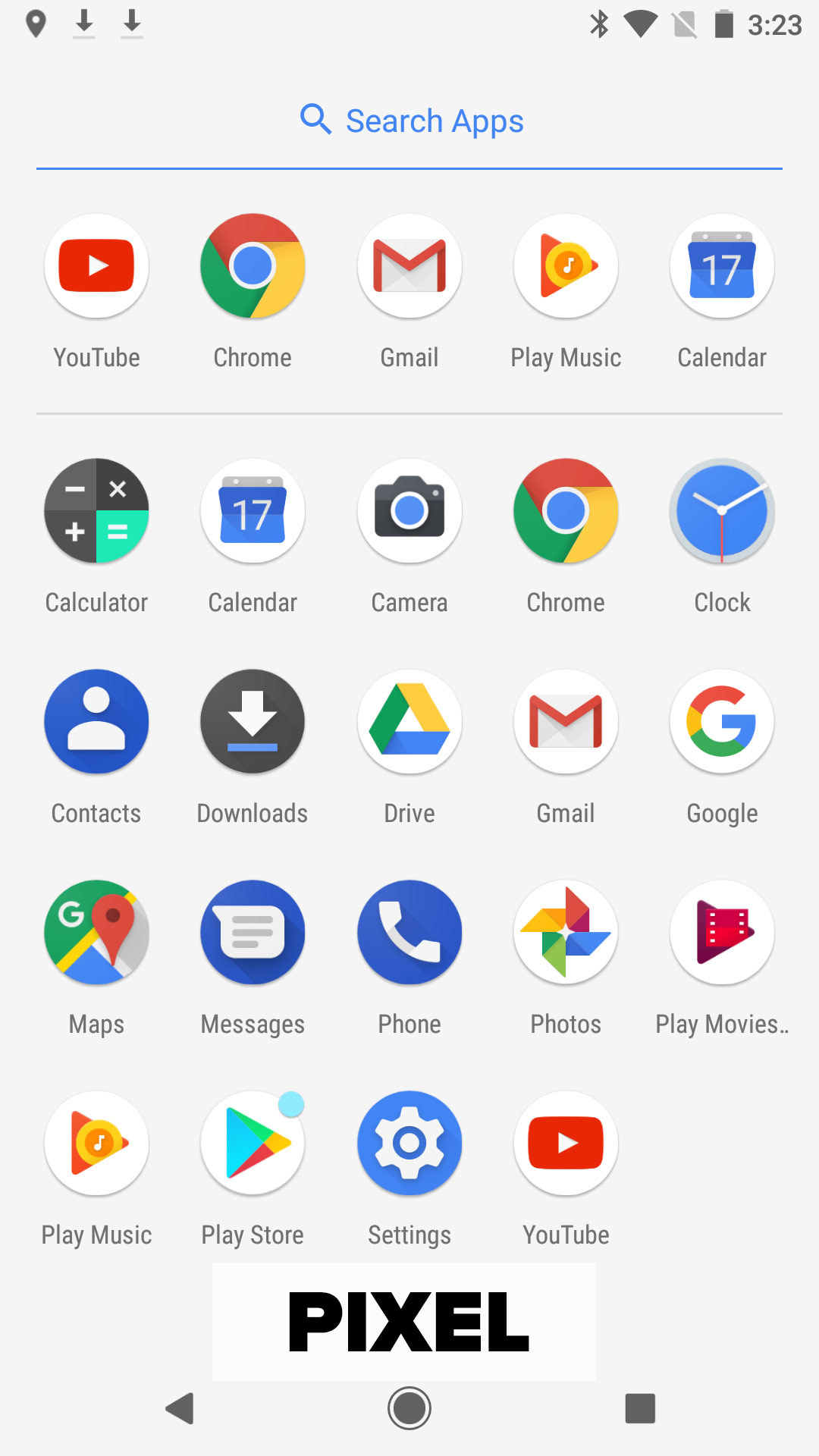This image is a screenshot of a smartphone's app icon page. The page features a light gray background and contains a total of 24 app icons neatly arranged in a grid format. There are five icons per row, except for the bottom row, which has only four icons, leaving a gap in the last column. 

At the top of the screen, there is a light blue rectangular bar with the text "Search apps" in the center. Next to it, on the left, is a blue magnifying glass icon, indicating a search function. Below this bar, the app icons are organized into rows and columns.

Each app icon is enclosed in a circular background, with the app's name written directly below its icon. The icons include recognizable apps such as YouTube, Chrome, Gmail, Play Music, and Calendar, among others. For instance, the Gmail icon prominently features its well-known red "M" design over a white envelope. 

At the bottom of the screen, in bold black capital letters, is the word "PIXEL" inside a very light gray rectangle, providing a subtle contrast against the screen's background color. This text likely indicates the brand or model of the phone.